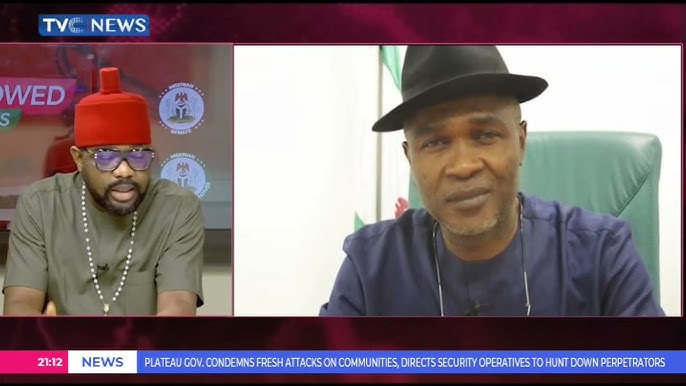In this horizontal screenshot of a news program on TVC News, the left side features a man donning a green t-shirt, white rosary beads, and a red cap. He appears to be sitting in a studio background adorned with various logos, possibly indicating he is a newscaster. Behind him, the TVC News logo can be seen prominently. To the right, seamlessly adjoining the left image, is a man in a blue cotton shirt with glasses around his neck, gazing quizzically at the viewer. He is seated in a green chair and is sporting a black top hat. A strip of text runs along the bottom of the image, featuring a pink, white, and blue color scheme. The text reads: "2112 News. Plateau Government condemns fresh attacks on communities, directs security operatives to hunt down perpetrators."